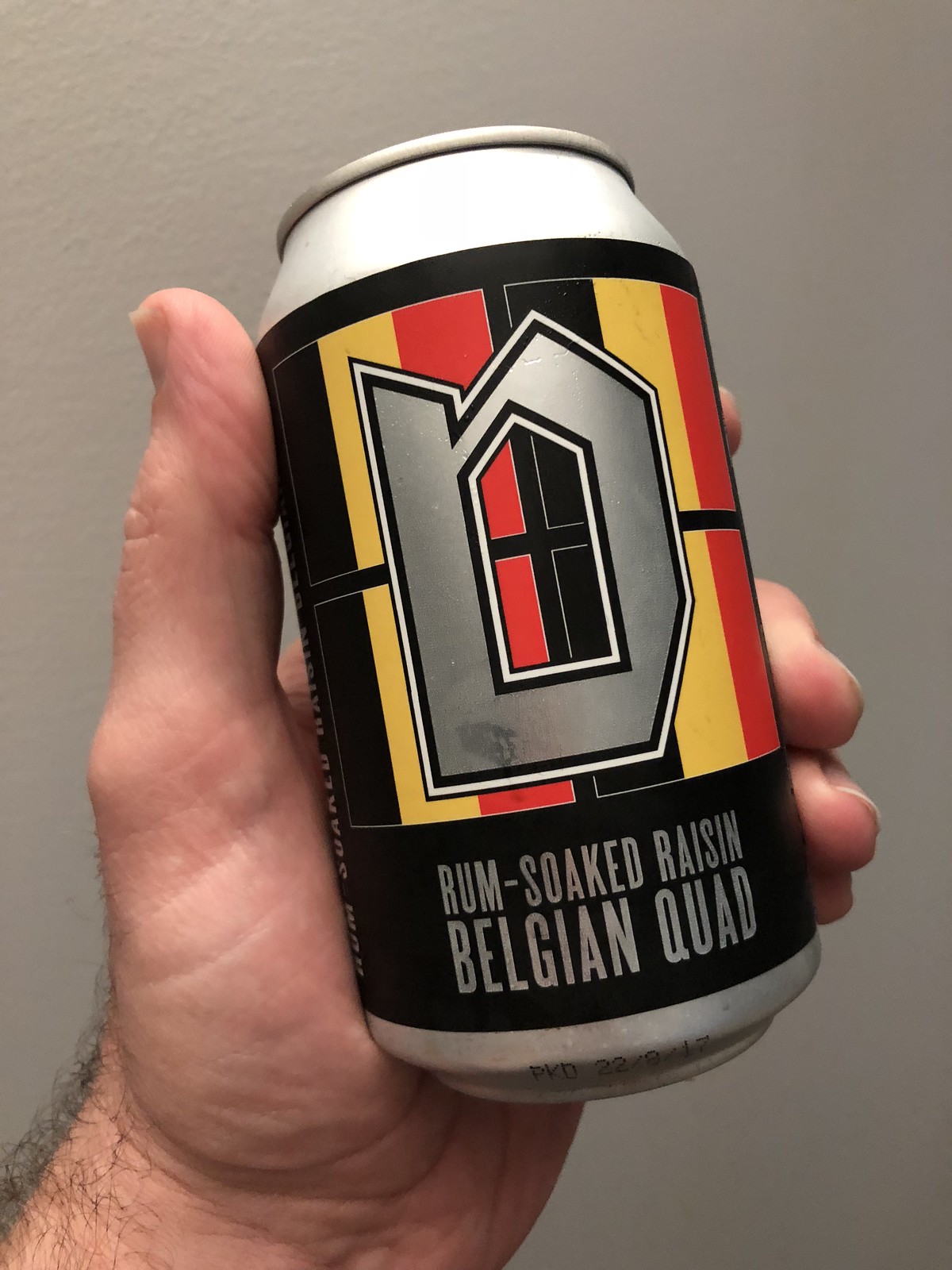In this image, a male left hand is prominently featured against a solid gray background. The hand, with the thumb positioned on one side and fingers wrapped securely around it, is holding a silver can. The can's design is striking, with a black label that prominently displays a giant silver "D" at its center. Behind this "D," there appears to be a window flanked by striped curtains in black, yellow, and red hues. The label at the bottom of the can reads "Rum Soaked Raisin Belgian Quad" in sleek silver lettering. The can is tilted at an angle, obscuring the top, leaving it unclear whether it is open or closed.